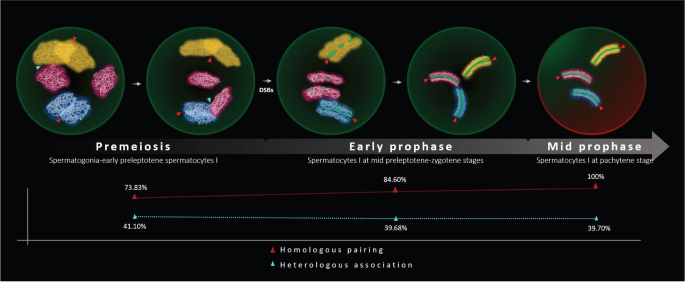The image is a detailed scientific diagram illustrating the dynamics of homologous chromosome pairing and heterologous association from spermatogonia to pachytene spermatocytes in Mus musculus (mouse). It presents a series of five circles at the top, each representing different phases of meiosis labeled as Pre-Meiosis, Early Prophase, and Mid-Prophase. The circles contain various colored blobs—yellow, blue, and garnet (appearing as purple)—which symbolize different homologous chromosomes. In some circles, green and red colors indicate the presence of TRA-98 and H1T, respectively.

The arrangement and interaction of these blobs change through the stages, depicting the pairing sequences. Homologous pairing is marked by a red arrowhead, while heterologous association is marked by a blue arrowhead. The green dotted or continuous filaments in the circles represent the SYCP3 protein. The bubbles show progress percentages: 73.83% in red, 84.50%, and 100% in different phases for homologous pairing, with a green line indicating heterologous association percentages of 41.10%, 39.68%, and 39.70%. The background of the diagram is predominantly black, enhancing the visibility of the colored structures within the bubbles.